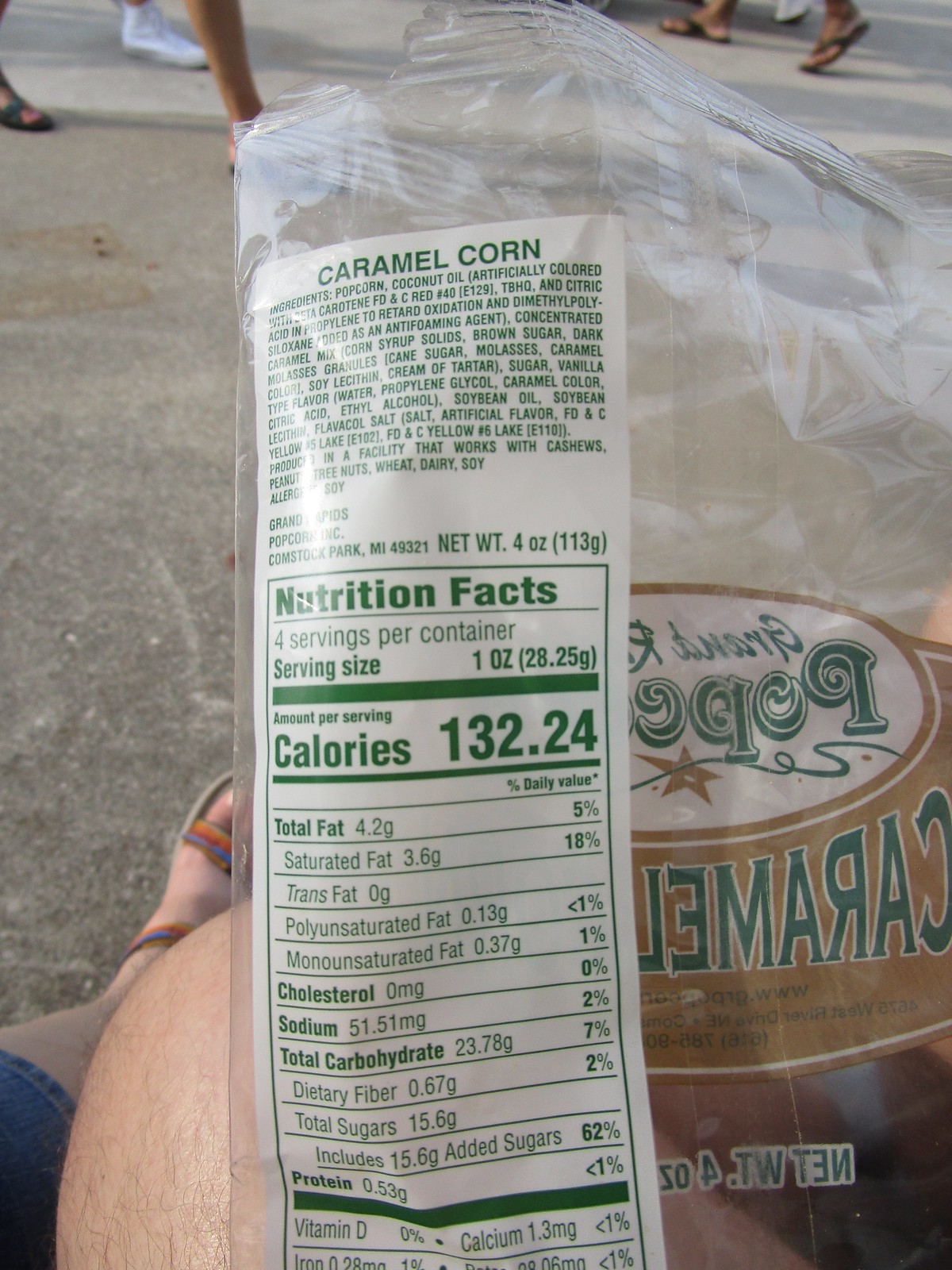The photograph depicts the back of an empty caramel corn package held on someone's lap. The nutrition label is prominently displayed with green lettering. On the left side of the image, the package details the ingredients and nutritional facts, including prominently featured calorie information with a total count of 1324 calories for the entire package, with each serving size being one ounce and a total of four servings per container. The word "caramel" is notably visible but mirrored, appearing backwards on the right-hand side of the image. In the lower section of the frame, part of the individual's knee and foot is visible; the foot is clad in a sandal, and the person is wearing three-quarter length denim pants.